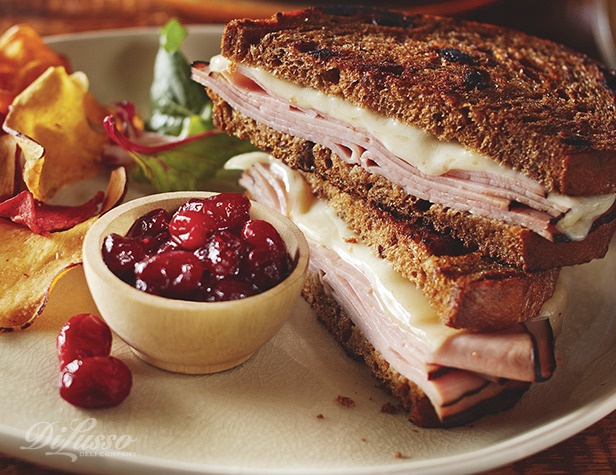The image features a detailed, close-up view of a lunch plate set on a brown wooden table. Dominating the right side of the circular white plate is a sandwich, likely made from dark brown or raisin bread, cut into two triangles and stacked on top of each other. The sandwich showcases visible layers of ham and melted white cheese. On the left side of the plate sits a small, round bowl filled with glazed or candied cherries, with a few cherries placed beside the bowl on the plate. Positioned behind the cherries, a mix of yellow, green, and red veggie chips can be seen, along with a small leaf of lettuce. The scene is styled in a photographic realism manner, emphasizing the textures and colors of the food. The background surrounding the plate is softly blurred, drawing more focus to the food arrangement. Notably, in the bottom left corner of the plate, partially hidden under the bowl, is a white script logo or photo credit that appears to read "DeLuso Deli Company."